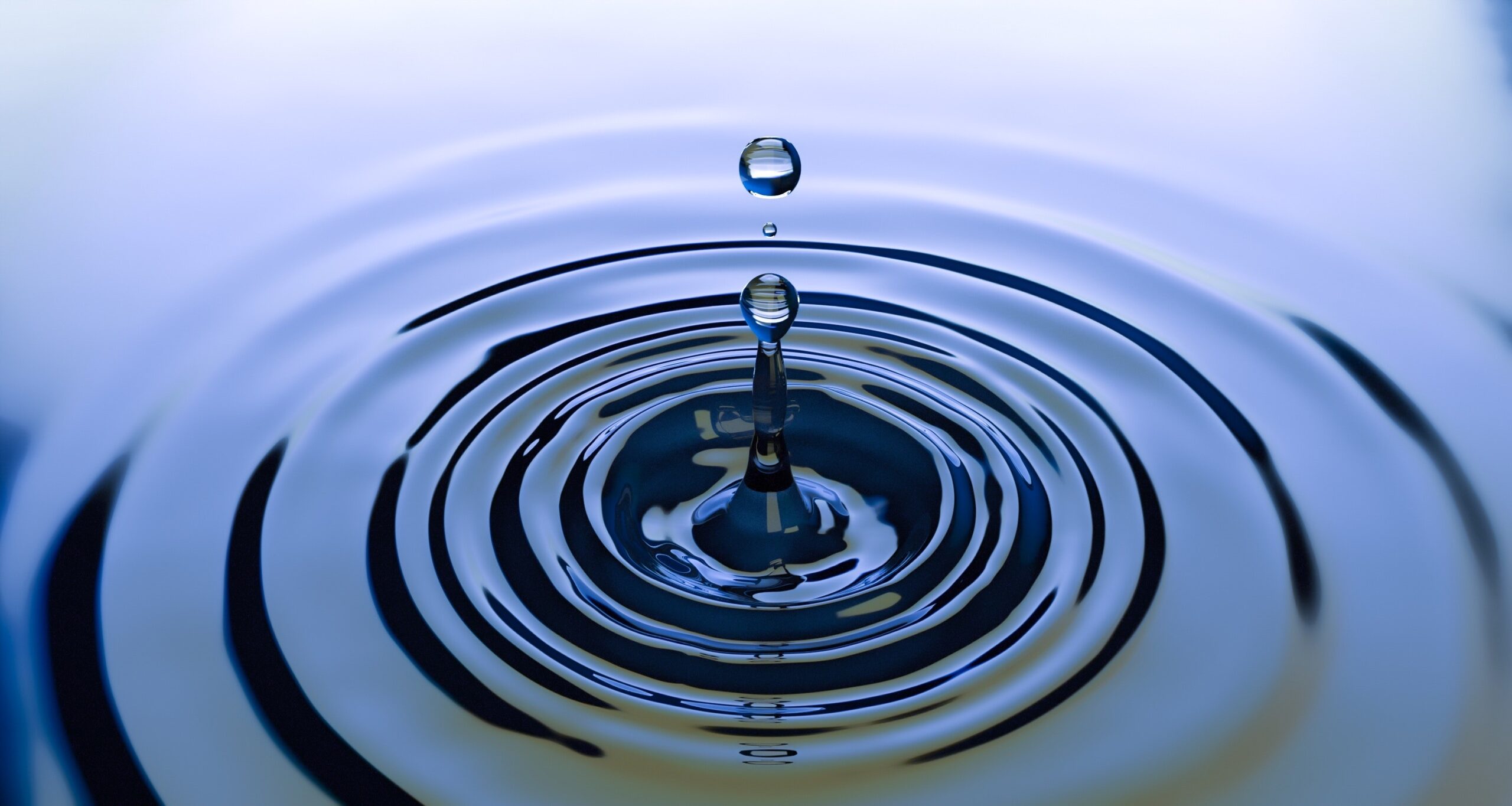A high-resolution, close-up image captures the precise moment a water drop hits a larger body of water, creating a dynamic ripple effect. At the center, the water forms a slightly sunken depression surrounded by a conical splash that ejects droplets upward. The impact suggests the drop fell from a significant height or had substantial weight, as evidenced by the thick, outward-moving ripples. The water's color transitions from a white hue in the background to a deep bluish-gray and then to a muddy green towards the image's bottom, conveying a sense of depth. The droplets suspended in the air appear pristine and transparent, magnifying the clarity of the water. Light reflections add a silverish tint, enhancing the visual appeal. The main action is frozen in time, emphasizing the interplay between the water drop and its larger aquatic environment.